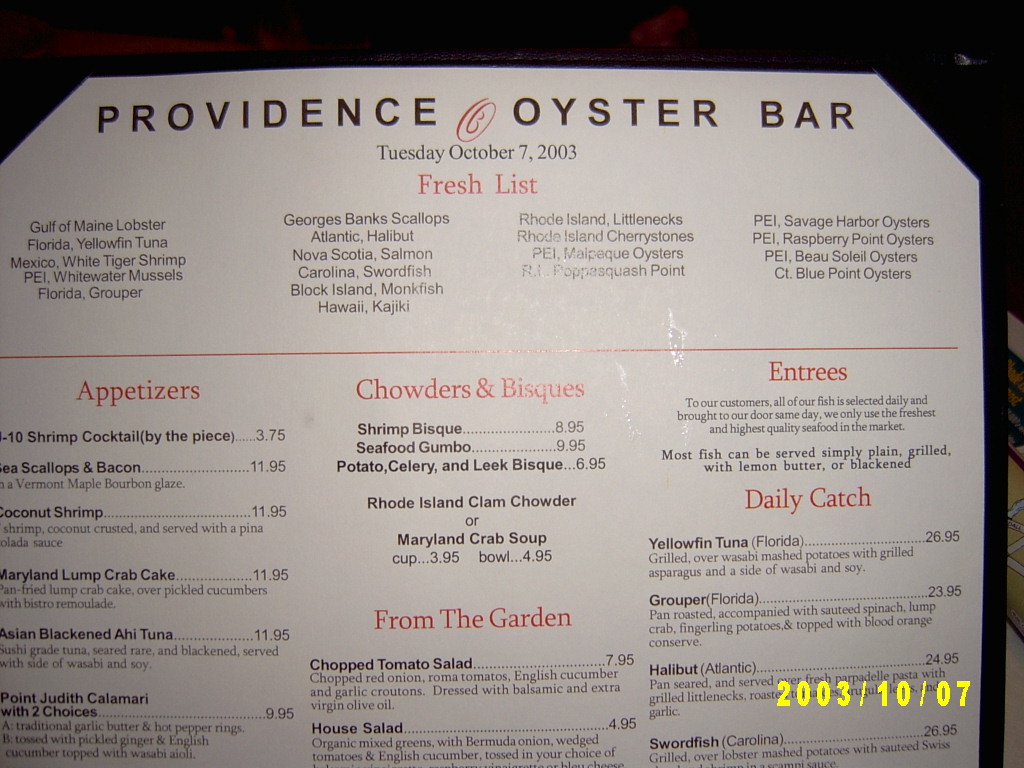This image features a snapshot of a menu from Providence Oyster Bar, encased in a sleek black frame with black corners at the top. The photograph captures only the upper portion of the menu page, which is printed on a cream-colored background with a mix of red and black text. 

In the lower right-hand corner, the date "2003-10-07" is superimposed in yellow, corresponding with the menu's date, "Tuesday, October 7, 2003", displayed at the top of the page.

Below the date, the heading "Fresh List" is prominently featured in red text, listing an array of seafood delicacies: Gulf of Maine lobster, Florida yellowfin tuna, whitewater mussels from Prince Edward Island, Atlantic halibut, Black Island monkfish, Rhode Island little necks, Rhode Island cherry stones, and three types of oysters from Prince Edward Island.

The menu is further divided into several sections, each labeled in red: "Appetizers," "Chowders and Biscuits," "From the Garden," "Entrees," and "Daily Catch." The "Appetizers" section includes items such as shrimp and crab cakes. "From the Garden" offers various salads. The "Daily Catch" section features four different species of fish. The text within each section is in black, maintaining a clear and elegant presentation.